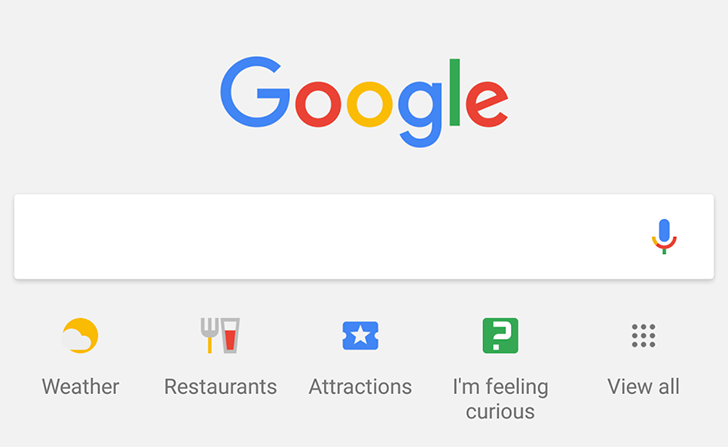The image depicts the Google homepage, known for its minimalist design, predominantly featuring a white background. Centered towards the top is the iconic Google logo, displayed in a large, bold font. The logo's letters are color-coded: the first 'G' is blue, the first 'O' is red, the second 'O' is yellow, the 'g' is blue, the 'l' is green, and the 'e' is red.

Beneath the logo, there is a search bar accompanied by a microphone icon on its right, symbolizing the voice search functionality.

Below the search bar, there are several icons representing various functionalities. Each icon is vividly colored and comes with a descriptive label:
1. A yellow circle featuring white cloudy details with the label "Weather" underneath.
2. A magnifying glass icon and a fork, indicating "Restaurants".
3. A blue square with a central white star, labeled "Attractions".
4. A green square with a white question mark, captioned "I'm Feeling Curious".

Additionally, towards the right, there is a grid of nine dots arranged in three rows of three. This grid acts as a menu, labelled "View All".

The polished and user-friendly design captures the essence of Google's commitment to simplicity and functionality.